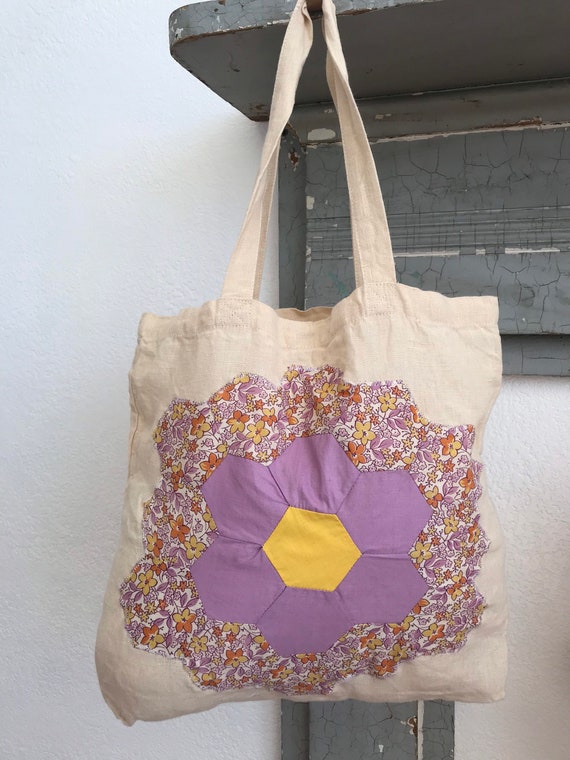A photograph showcases a detailed canvas tote bag hanging from an old, gray, and cracked wooden shelf. The shelf, which features an ornate yet weathered design, is mounted on a white wall. The vertically aligned image emphasizes the shelf at the top, from which a hook suspends the tote bag. 

The tote bag, beige in color and made of cloth fabric, features two handles and appears to contain items, indicating it is not empty. The central design on the bag is a striking patchwork flower composed of hexagonal fabric pieces. The flower's center is a bright yellow hexagon, surrounded by purple hexagon petals. This central flower is framed by an intricate border of smaller, cartoonish flowers in yellow, orange, and purple, forming a ditzy floral pattern that covers much of the bag’s front.

Together, the weathered gray shelf and the colorful, patterned tote bag create a harmonious contrast against the clean, white background, capturing a blend of rustic and whimsical charm.